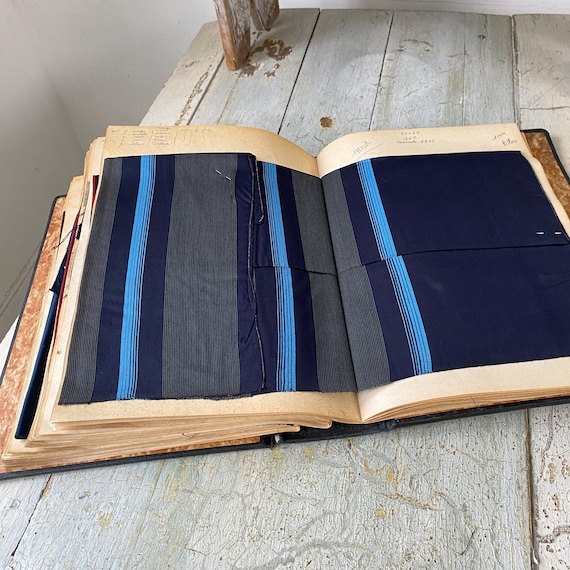An overhead and slightly angled view reveals an old, rustic book lying open on a rugged, white wooden table, which is chipped, dusty, and bears visible scratches. The table, positioned against a whitish-gray wall matching its aged appearance, enhances the rustic scene. The book itself has worn, beige pages and a black border around its edges, indicating its age and frequent use. The open pages display a piece of fabric, intricately stapled or attached, spanning across both left and right pages. This fabric has a striped pattern with colors ranging from dark navy blue to light blue and thick gray stripes. The cloth is arranged with alternating colors creating a sequence of thin and thick stripes, adding a textured depth to the pages. Despite the indecipherable writing on the pages, it appears the book serves as a historical fabric collection or a demonstration of old textiles, with other fabric pieces protruding slightly from the bulk of the remaining pages. The overall ambiance suggests a meticulous preservation of textiles, showcasing their historical significance in a visually compelling manner.